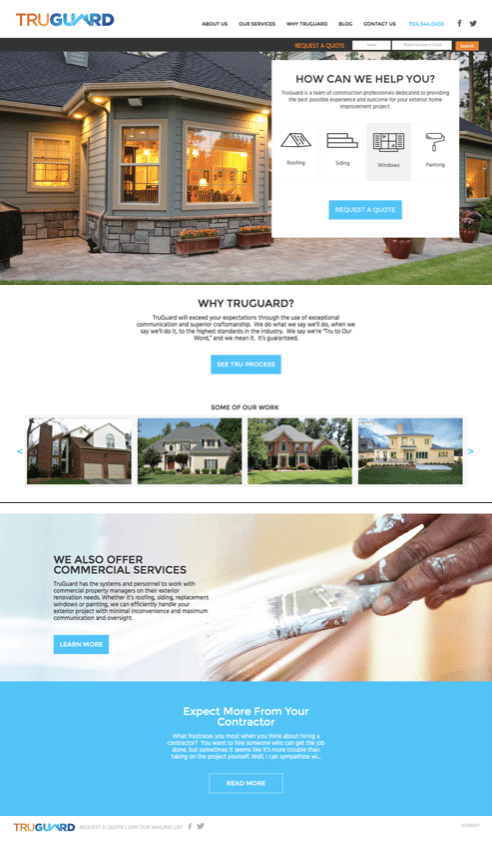TrueGuard TRU - Home Services Redefined

TrueGuard TRU boasts a clever logo where the 'A' in "Guard" is creatively designed to resemble the pitched roof of a house, emphasizing the company's dedication to home protection and improvement. At the top of the webpage, users will find easily navigable links to key sections: About Us, Our Services, Why TrueGuard, Blog, Contact Us, and a prominently displayed phone number for direct inquiries.

Dominating the screen is an inviting image of a modern, well-lit house at dusk. The warm glow from the interior lights contrast beautifully against the house's sleek grey exterior. Surrounding the home is meticulously maintained landscaping, with various plants artfully arranged around the perimeter.

Beneath this captivating image is the heading "Why TrueGuard," followed by a succinct but impactful promise in smaller text: "TrueGuard will exceed your expectations through the use of exceptional communication and superior craftsmanship." Nearby, a prominent blue button labeled "See True Process" invites users to learn more about the company's distinctive approach.

Scrolling further, the page showcases additional imagery of both residential and commercial services. Notably, there's a close-up shot of a professional painter at work, capturing a hand applying fresh white paint with a brush, symbolizing the quality and attention to detail TrueGuard TRU is known for.

Explore what sets TrueGuard apart and discover how their expertise can cater to both your residential and commercial needs.